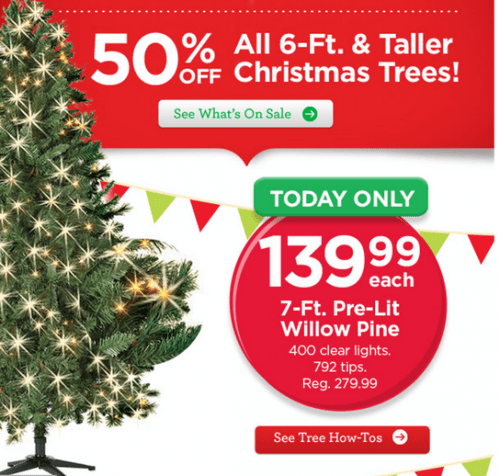Promotional Graphic for Christmas Tree Sale:

The promotional graphic showcases an exclusive sale offering 50% off on all Christmas trees that are six feet and taller. A prominently featured, beautifully illuminated pre-lit Willow Pine Christmas tree serves as the centerpiece of the graphic. The tree, adorned with 400 clear, twinkling lights, offers a warm, starry glow that contrasts its deep green foliage. With 792 tips, it provides a lush and full appearance perfect for the holiday season.

Highlighted in the graphic is a special "Today Only" offer, pricing the seven-foot pre-lit Willow Pine tree at $139.99 each, down from its regular price of $279.99. This exceptional deal is boldly noted against a festive background, with vivid holiday-themed elements. The background primarily features a clean white color, accented with bright red holiday motifs and vivid green banners, creating a festive and inviting atmosphere. The sale detail text is crisp white, ensuring clear readability.

A clickable button labeled "See Tree How-Tos" is positioned at the bottom of the graphic, inviting customers to explore detailed instructions and tips for setting up their newly purchased Christmas tree. The overall design effectively combines informative content with eye-catching visual elements, making it a compelling and engaging advertisement for the limited-time Christmas tree sale.